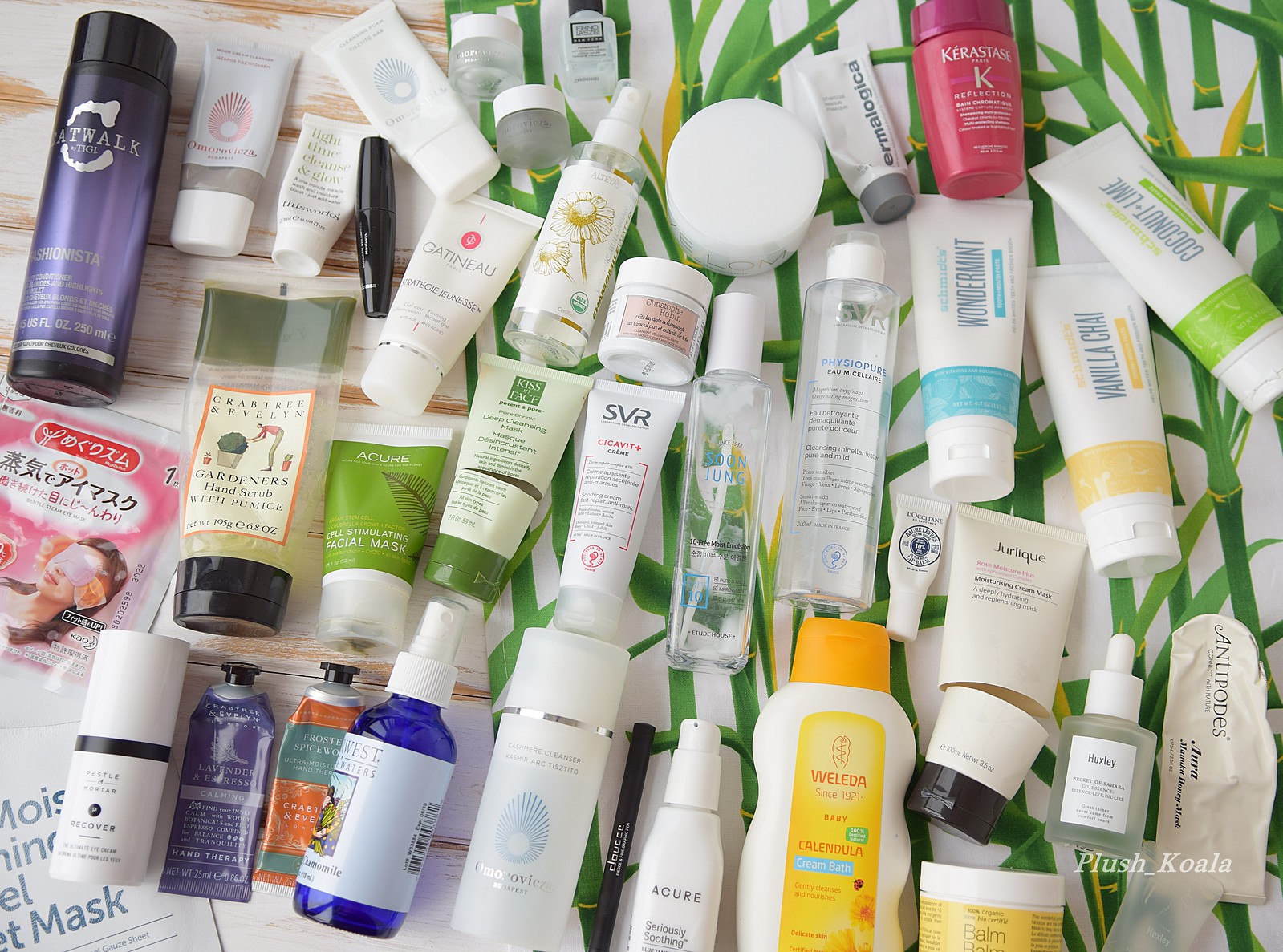The photograph depicts an orderly array of travel-sized and sample-sized bottles and jars, meticulously arranged on a dual-patterned surface. The main section of the background features a predominantly white surface with subtle green streaks reminiscent of grass or corn blades. To the left, another cloth-like surface with a white background is adorned with horizontal, round streaks. 

The selection of containers includes a variety of small, capped tubes and bottles, many of which are too small to decipher. The bottles and tubes are primarily white, adding to the uniformity of the display. 

In the upper right corner of the arrangement, there are several legible items: a striking red or hot pink terraced bottle resembling a shampoo container; beneath it, a white bottle with an aqua banner reading "Wonder Mint"; and to the right, three white tubes each distinguished by the colored borders around their caps—one with a yellow border labeled "Vanilla Chai," another with a lime green border labeled "Coconut Lime."

In the immediate foreground, near the center of the display, a distinctive white, curvy-sided bottle with a yellow cap and label features the names "Lolita" and "Calendula." Above this, two slender, clear bottles are placed, adding to the assorted collection.

There are approximately four rows of these items, though they are closely packed together. In the upper left corner, a metallic purple bottle labeled "Catwalk" stands out, potentially a sample bottle. Below this, a pink-labeled eye mask adorned with what appear to be Chinese characters is visible.

This diverse assortment includes a lime green bottle in the middle, further adding to the variety, and numerous other items, creating a visually engaging array of travel-sized personal care products.